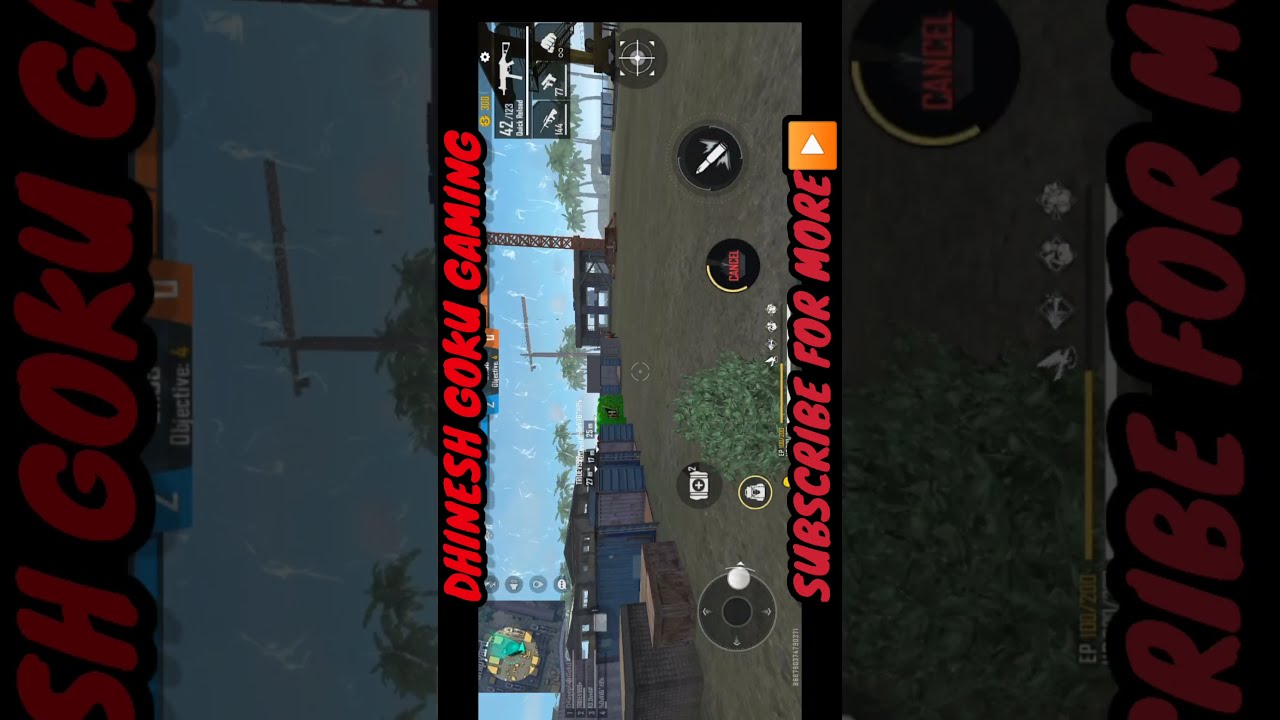The image is a wide rectangular composition depicting a sideways screenshot of a YouTube gaming video. In the center, an outdoor video game scene shows a bright green bush surrounded by green grass, blue and gray buildings, and palm trees in the background. Large cranes and a construction zone with crates are visible, indicating elements common in a first-person shooter game. Left and right of this central screenshot are darker, close-up fragments of the same image, creating a layered effect. The image includes a visible heads-up display (HUD) typical of video games. In bold red font at the top, it reads "Dinesh Goku Gaming," and at the bottom, "subscribe for more."